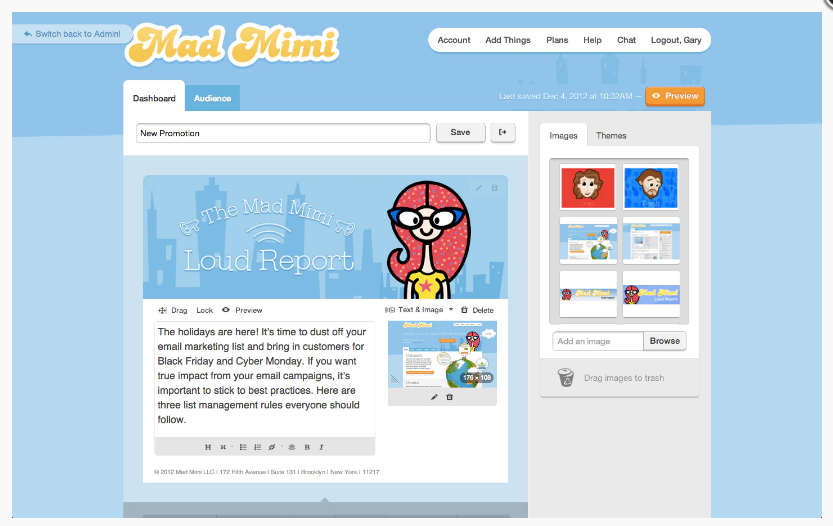This is a screenshot of the Mad Mimi website interface, specifically displayed on Gary's account. The interface features several key components and functionalities described in detail.

On the top-left corner of the screen, there's an option to switch back to the admin view, highlighted in light blue, with the words "switch back" in a darker blue tone. Adjacent to this, you'll find sections labeled as Account, Add Things, Plans, Help Chat, and Log Out, confirming that Gary is currently logged in. These options are displayed in black text within a long, white, oval-shaped bar.

Beneath the main Mad Mimi header, which is presented in yellow, there are several tabs, with "Dashboard" being the active tab. Below this, there is a section promoting a new campaign titled "Mad Mimi Glad Report." This section features a cartoon image of a woman with distinctive black eyes, blue glasses, and long red hair. She is wearing a yellow shirt adorned with a red star in the center.

The interface provides interactive options such as dragging, locking, or previewing the campaign content. It includes a description encouraging users to update their email marketing lists ahead of the holiday season, emphasizing best practices for effective email campaigns. Key dates mentioned include Black Friday and Cyber Monday.

On the right side, there is a preview pane displaying how the webpage will appear to recipients. Directly beneath the "Log Out Gary" button, an orange "Preview" button is positioned. This is followed by two tabs: Image and Theme. The Image tab is currently active, showcasing six different images with an option to add more images. There's also a search field available for locating specific images.

Overall, this screenshot offers a comprehensive view of the various functionalities and visual elements present on the Mad Mimi email marketing platform, demonstrating its user-friendly and visually distinct interface.